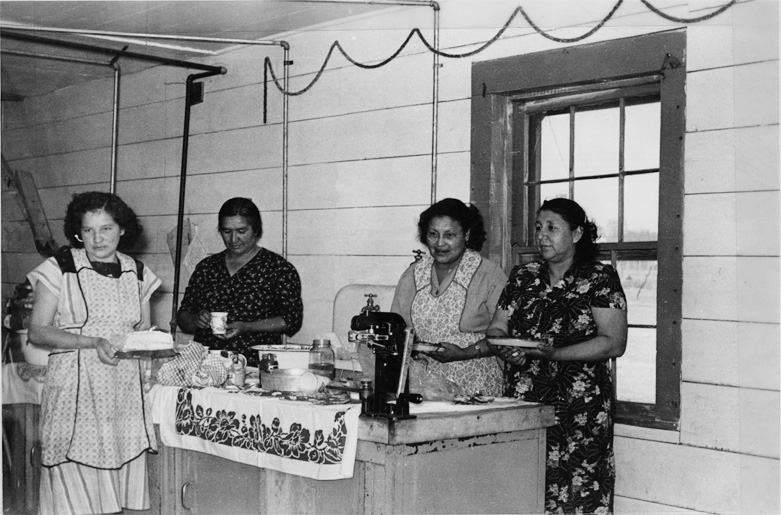This black-and-white photograph captures four middle-aged women with dark, curly hair, standing behind a countertop, seemingly engaged in cooking or meal preparation. Each woman is holding either a plate, platter, or cup, likely containing a baked good or another culinary item. The countertop they stand behind is adorned with a decorative cloth and features various kitchen tools, including a mixer-style machine.

From left to right, the first woman is wearing a striped white dress with an apron over it, and she appears to be holding a cake. The second woman is dressed in a black and white polka dot top, while the third woman, donning a white speckled apron, is positioned next to her. The woman on the far right, wearing a floral dress, holds a platter. They are situated within what appears to be a kitchen or a house, characterized by a white panel wall, exposed pipes, and wires above them, along with a wooden windowsill and standard wooden window behind the two women on the right. The image, despite its limited detail due to the lack of color and clarity, provides a nostalgic glimpse into a communal cooking scene.